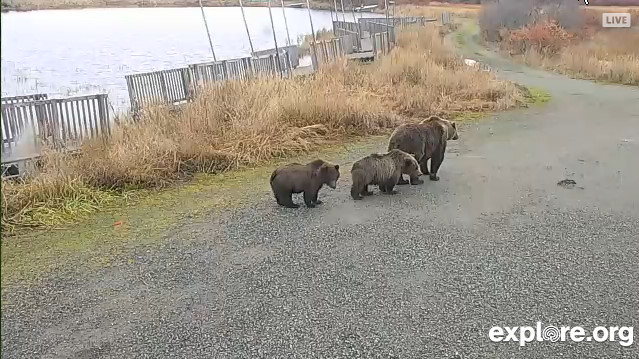This photograph captures a serene outdoor scene focused on three black bears walking along a gravel road. The road, which starts in the foreground and curves to the right before bending to the left, appears to become smoother as it extends into the background. Leading the small parade is a larger bear, likely the mother, followed closely by two smaller bears, possibly yearlings. Their sleek, dark fur contrasts with the light gravel beneath them.

In the bottom right corner of the image, the text "explore.org" is visible, indicating that this is a live-streamed broadcast, which is confirmed by the "LIVE" label in the top right corner. To the left of the road, the landscape features a mix of wheat-colored and brown seagrass, suggesting a summer setting, with patches of green grass interspersed. This plant life resembles the kind found near coastal areas.

Beyond the seagrass, there is a gray wooden fence, which parallels a pathway reminiscent of a boardwalk leading towards the water. The water itself, visible on the left side, is a light blue color with gentle waves, evoking a peaceful, natural environment. Scattered in the background are small docks and walkways, which contribute to the overall tranquil, waterfront ambiance of the scene.